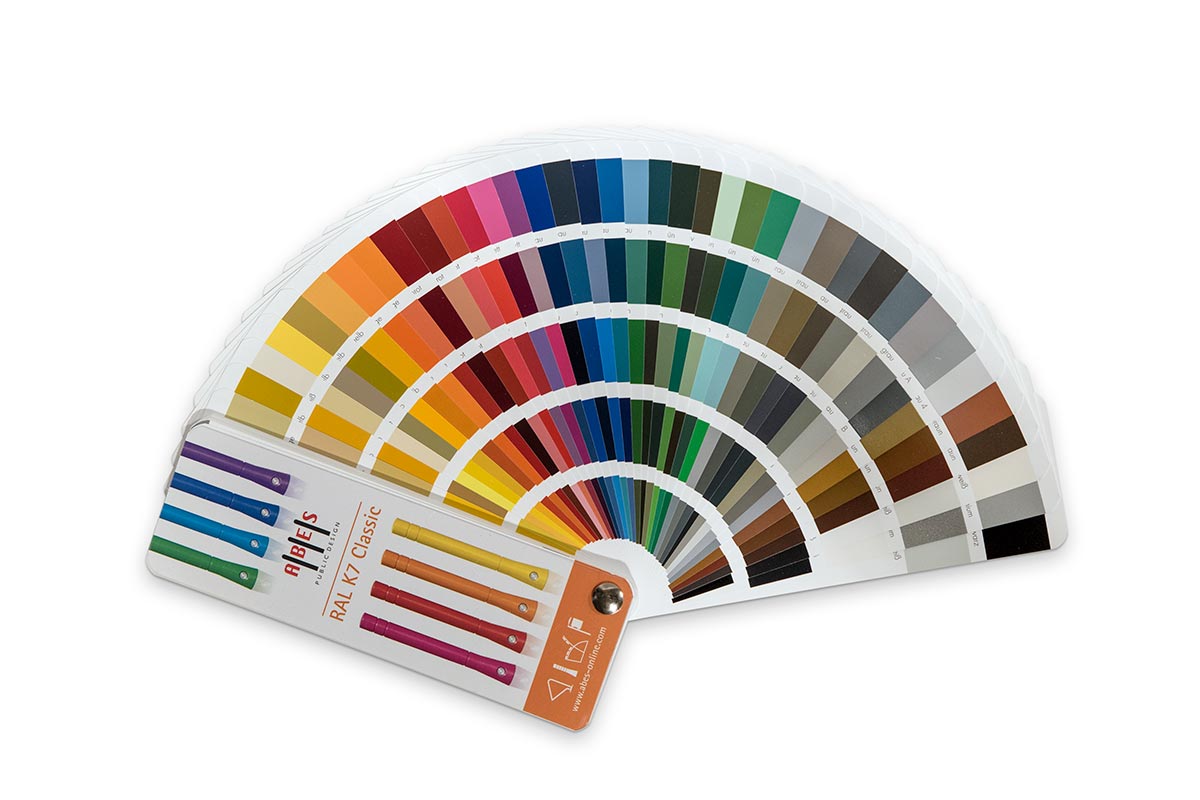The image depicts a partially fanned-out color wheel featuring a broad spectrum of hues, arranged logically from golden yellows to shades of yellow, orange, red, pink, dark and light blues, greens, turquoise, tan, brown, white, gray, and silver. The color wheel is laid against a white background, and not all shades are fully visible due to partial fanning. On the left side of the color wheel, there is a rectangular case with white and orange accents, labeled "R.A.L. K7 Classic." The case also displays an image of paint pens in a gradient ranging from pink to yellow.